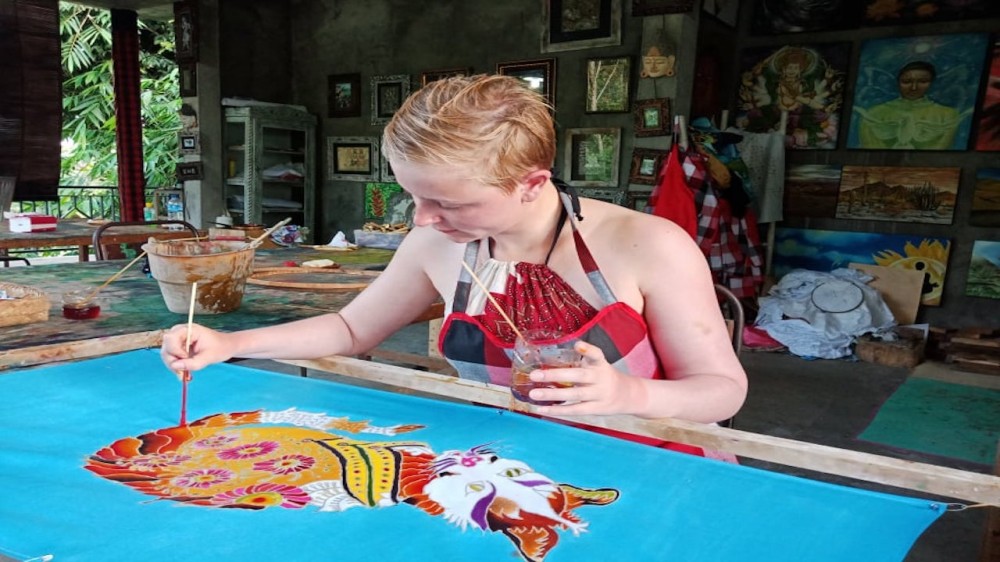In a well-lit workshop room with brown walls and windows in the background, a young woman with naturally red hair sits at a slightly cluttered wooden table, immersed in her painting. She is dressed in a paint-splattered smock and holds a brush in her right hand and a small glass, possibly containing a drink, in her left. The table is covered with various painting supplies, including a bucket of paint. On the table before her is a wooden frame holding a vibrant blue canvas, upon which she is painting a colorful cat adorned with intricate designs in red, pink, yellow, and light blue, with detailed orange and pink flowers, as well as trees in the background. The artist is captured in mid-action, her focus entirely on the work, creating a lively, detailed piece that fills the central frame of the photograph.